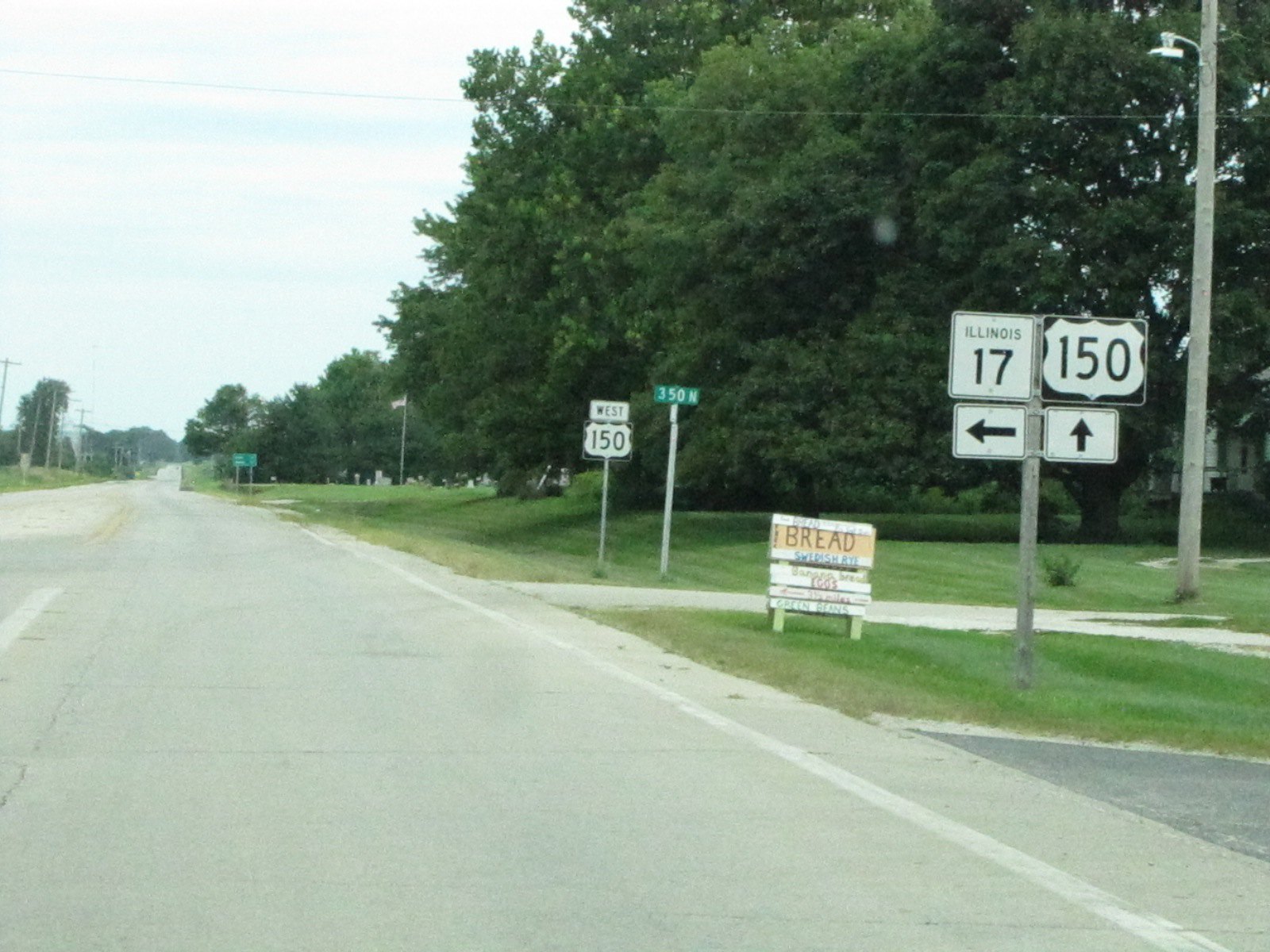The image depicts a concrete road, which seemingly splits in the middle evidenced by a barely visible white line, offering a perspective that narrows as it extends into the distance. The right side of the road is lined with dense, lush green trees. Adjacent to the trees on the right, there's a metal pole with a complex black and white sign featuring multiple directives: "Illinois 17" and "150," with arrows pointing left and straight, respectively. Below, there's a small wooden sign bearing the word “Bread,” along with a street sign labeled “350.” Further down, a smaller sign reads "150 West."

In the diminishing distance, obscured by perspective, an American flag is perched atop a tall pole, paired with a green sign whose text is illegible. The left side of the road is largely empty, populated by a few scattered trees in the far background. The sky can be seen in the upper left corner of the image, extending slightly towards the middle.